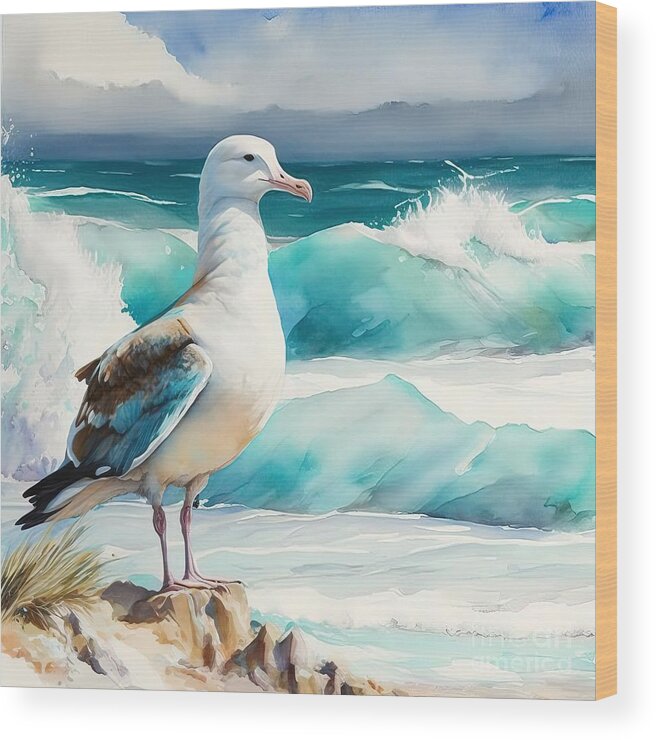This detailed painting captures a serene outdoor scene featuring a solitary white seagull perched on a small rock amidst a vibrant coastal environment. The seagull, facing right, has closed wings with intricate markings of blue, brown, and hints of darker brown or black at the tips. Its beak is a delicate light pink, and it stands on pink talons, with a single small black beady eye visible. Behind the bird, the clear aquamarine blue ocean displays large waves crashing into the shore, while the cloudy sky above, cloaked in gray with just slivers of blue peeking through, hints at an impending storm. The painting employs a beautiful palette of light blues, whites, and grays to depict the dynamic interplay of water and sky. Notably, in the bottom right corner of the wooden-edged canvas, there's a watermark, partially legible, with the word "America" visible, suggesting this might be an online catalog or artwork description. The seagull appears to be bracing itself against the wind, adding a sense of movement and life to the scene.